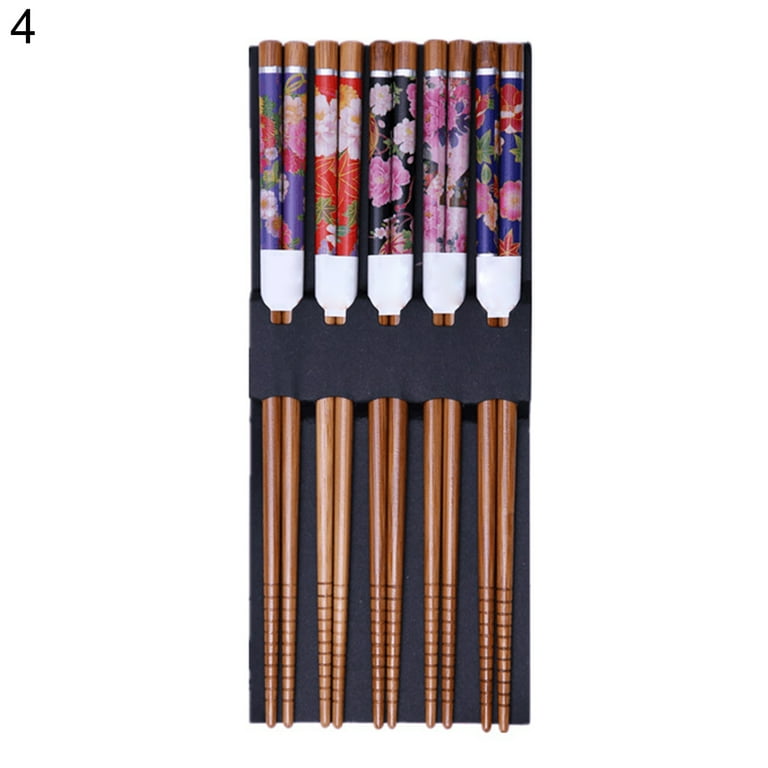In the stark white background of the image, a set of five ornately designed chopsticks are the sole focus, neatly arranged in a sleek, black holder. This holder grips the chopsticks around their midsections, showcasing the distinct and intricate designs of the handles as well as the textured, notched ends intended to hold food securely. The beautifully decorated handles vary in color and pattern, with floral motifs lending each chopstick a unique appearance: from left to right, the designs include a purple handle with flowers, a red handle with white flowers, a black handle with pink and white flowers, a pink handle with pink and black flowers, and a blue handle with red and pink flowers. The chopsticks are made of the same wooden material, with subtle variations in wood color, ranging from lighter to darker shades. The arrangement suggests a product display, possibly from a catalog, with a small number "4" visible in the upper left-hand corner. The image exudes a sense of elegance and careful craftsmanship, emphasizing the reusable nature and aesthetic appeal of these decorative chopsticks.